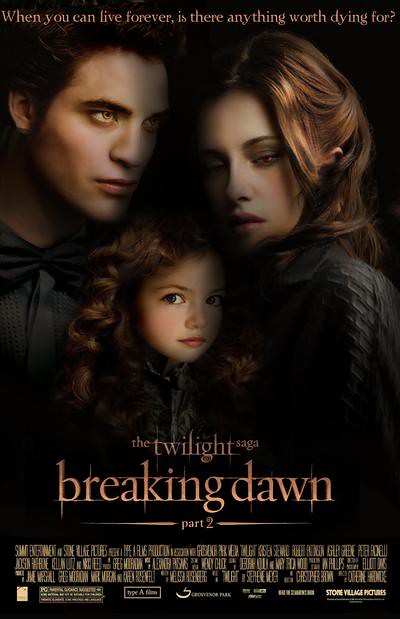This image is a movie poster for "The Twilight Saga: Breaking Dawn Part 2." The entire poster has a dark, almost black background that gives it a somber and intense atmosphere. In the center, there are three main characters: a serious-looking man (Edward) at the top, gazing slightly upward; a young woman (Bella) with brown hair next to him, looking down with an intense expression; and a young girl (Renesmee) with brown curly hair in the center, looking straight ahead. The poster features a bronze and brown color scheme, giving it a dark, moody overtone.

At the top of the poster, the tagline reads, "When you can live forever, is there anything worth dying for?" This thought-provoking question sets the tone for the movie. Below the main characters, the title "The Twilight Saga" is displayed in a light gray or white font, followed by "Breaking Dawn" in a fancy, gold-like font with a slightly gothic style, and finally "Part 2" between two decorative bars.

At the very bottom, there are several lines of unreadable text, likely credits, along with various logos, all set against the black background. The overall design emphasizes the dramatic and intense themes of the movie with its strategic use of colors and positioning of characters.